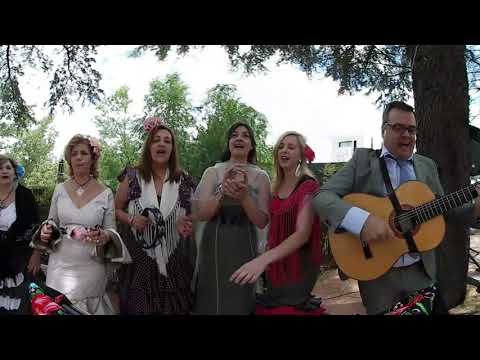In this outdoor scene, a musical troupe is performing under the shade of a tree, in what appears to be a park. The group consists of six people: one man and five women. The man, positioned on the right side of the image, is playing a guitar. He has glasses and is dressed in a grey suit with a white dress shirt and a light grey-blue tie. Behind him, there's a large tree trunk and some evergreen trees. 

To his left, five women are singing and holding tambourines. The woman closest to him is in a red dress, adorned with a red flower in her hair, and she's glancing downwards. Next to her is a woman wearing a light top and a whitish-green skirt. The third woman from the right is dressed in a dark grey dress with black stripes, possibly a white shawl, and her long hair falls over her shoulders. She also holds a tambourine. To her left stands a woman in a white dress with a necklace and blonde hair, accented by a pink flower. The woman furthest to the left, partially visible, has a blue flower in her hair, wearing a white top with what could be a black sweater. The sun is high in the sky, casting a soft light over the scene. The setting includes several trees and a building, suggesting a tranquil park environment.